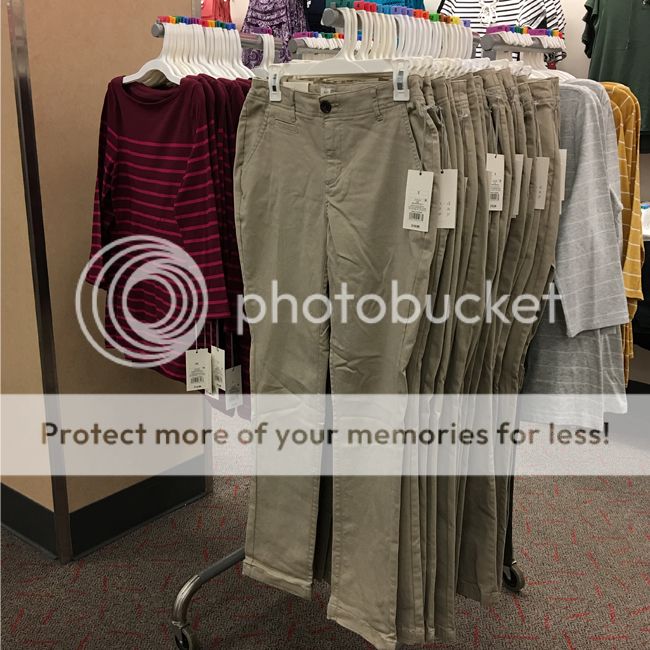This image depicts a clothing store scene centered around a prominent metal clothes rack filled with various garments. On the left side of the rack hang light beige khaki pants, neatly separated from an assortment of shirts displayed to the right. The shirts are of the same style but differ in colors—white, yellow, and plum with horizontal stripes. All garments are adorned with price and size tags and are hung on white hangers. In the background, additional shirts, possibly gray and orange polos, are hung on a yellow wall without clearly visible supports. The store's floor is covered in a brown carpet interspersed with red patterns. Dominating the image is a semi-transparent watermark featuring the "Photo Bucket" logo with multiple circles, accompanied by the phrase "Protect more of your memories for less" set in a white translucent banner. The overall setting suggests a department store environment designed for customer browsing.